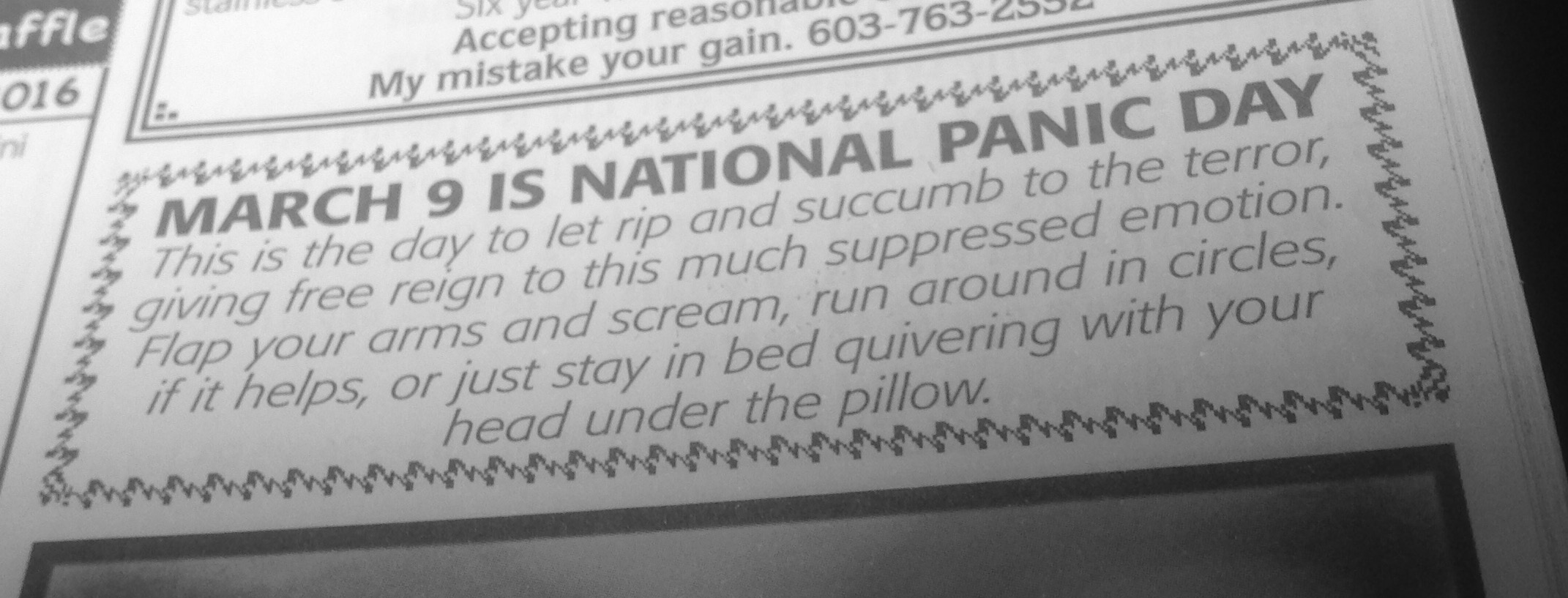This black-and-white photograph captures a section of an old newspaper or magazine. The highlighted text on a white background boldly announces in large capital letters: "March 9th is National Panic Day." This notable day is described as an opportunity to "let rip and succumb to terror," giving freedom to much-suppressed emotions. The accompanying smaller text suggests dramatic ways to embrace the day, such as flapping your arms, screaming, running around in circles, or staying in bed with your head under a pillow. The focal text is bordered by zigzag lines. Above the featured section, partially visible boxed ads tease with headlines like "My mistake, your gain," accompanied by a phone number, while additional ad boxes appear below.